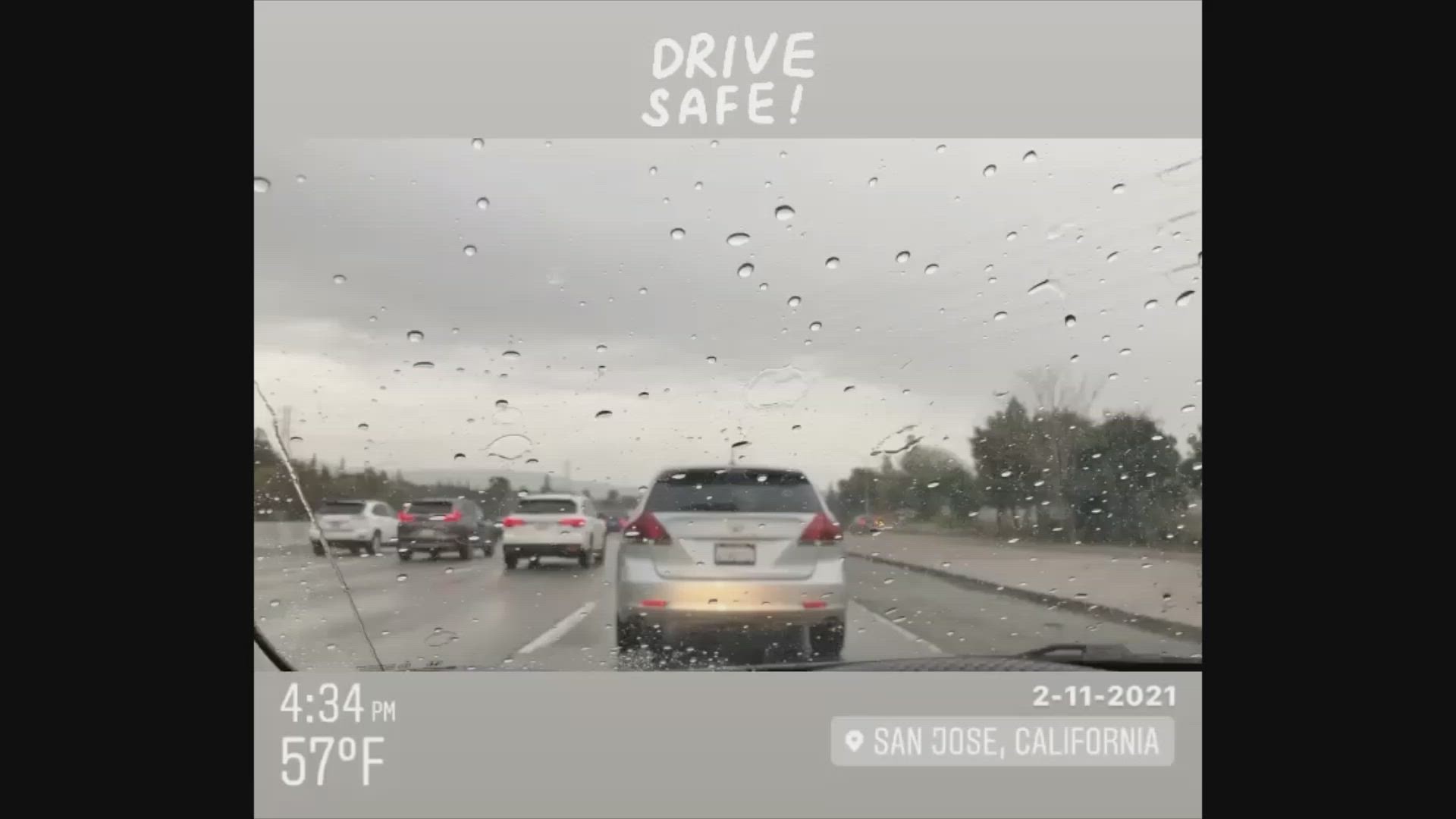A digitally created image features a cartoonish message at the very top in white text that reads, "Drive Safe." The scene is framed by two gray rectangles, one at the top and one at the bottom. The upper gray rectangle indicates the time as 4:34 PM, while the bottom rectangle displays the temperature as 57 degrees Fahrenheit. To the right side of the image, the date 2-11-2021 and location 'San Jose, Columbia, California' are listed.

In the main section of the image, a silver car is driving forward in the left-most lane. Adjacent to it, a white car occupies the next lane, followed by a black car and another white car in the subsequent lanes. The road is bordered by trees on both sides, showcasing green leaves that add a touch of nature to the urban scene.